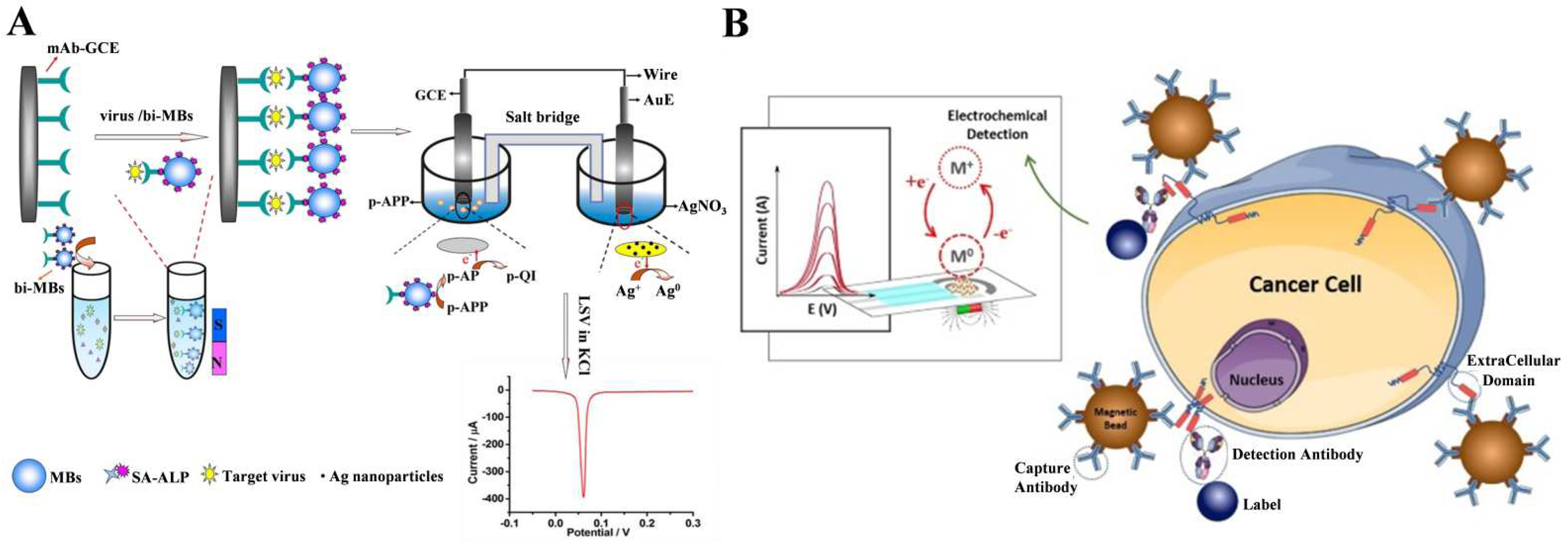This is a narrow, horizontal, rectangular scientific schematic about cancer, depicting the processes related to detecting and understanding cancer cells. The image is split into two halves labeled A and B. 

On the left side (A), the graphic includes intricate graphs and diagrams, with terms like "SALTBRIDGE" and various chemical symbols such as AUE, GCE, PAP, and AG. There are several drawn test tubes, likely representing an experimental setup, along with images that might depict viruses. The text includes phrases such as "MILSS AALP target virus particles."

The right side (B) is more medically focused and features charts related to electrochemical detection. Dominating this section is a large blue circle labeled "CANCER CELL," with a clear depiction of a nucleus. Surrounding the cancer cell are four smaller cells named "Extracellular Domain Capture Antibody." Below the large cancer cell, there is a section labeled "DETECTION ANTIBODY." Additional elements and labels like "Detection Antibody" are also present. A logo is placed at the bottom of the image. This schematic serves as an educational demonstration graphic intended for medical or scientific audiences.